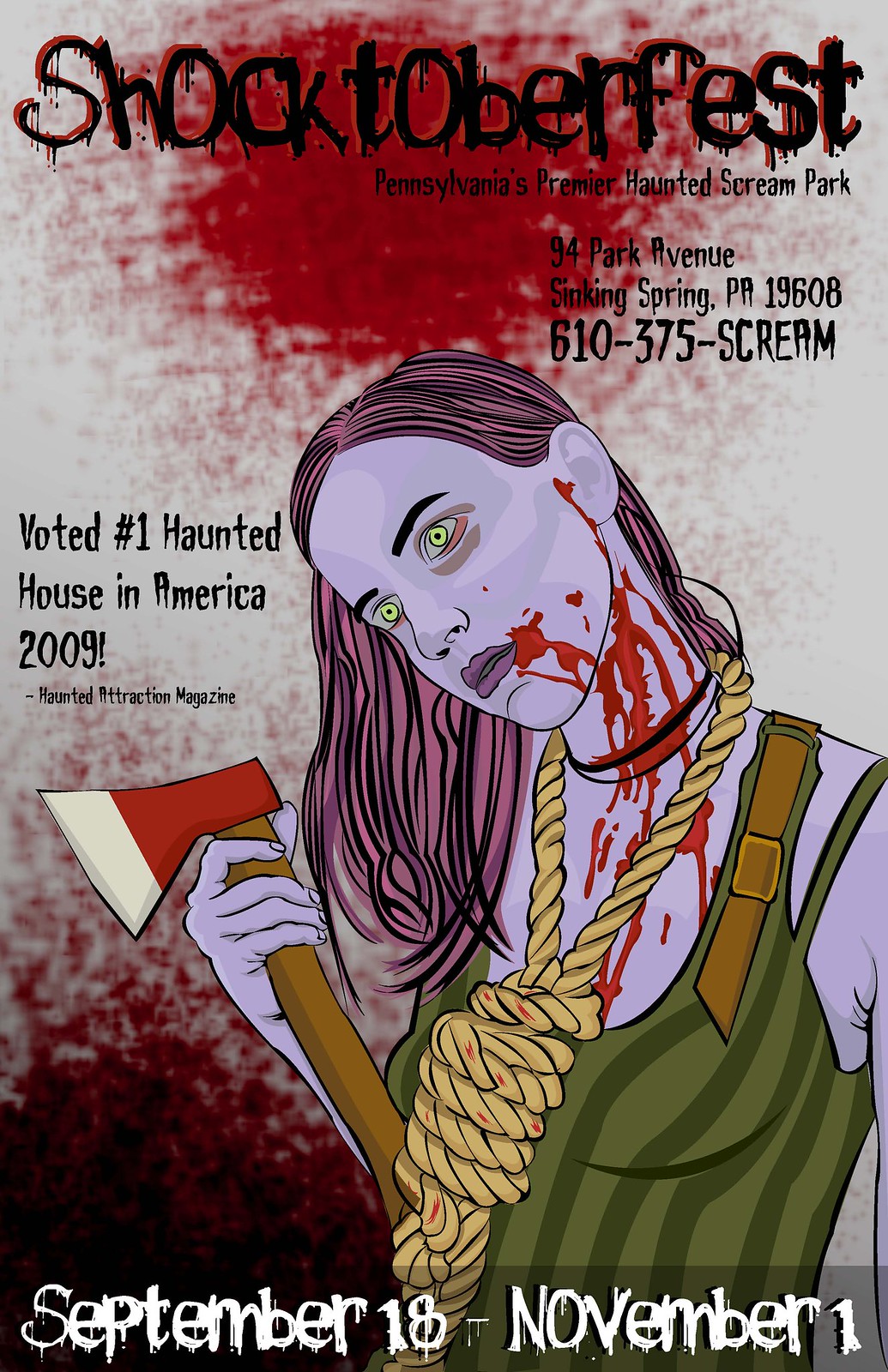The image is a detailed, eerie drawing designed as a promotional poster for "Shocktoberfest," Pennsylvania's Premier Haunted Scream Park. The background of the poster is grey, with large, dark red blood splatters at the top center and bottom left. Across the top, in black, haunted text that appears to be bleeding, the word "Shocktoberfest" is prominently displayed, with smaller text below announcing "Pennsylvania's Premier Haunted Scream Park."

The poster's central focus is a striking drawing of a female zombie with purple skin. Her appearance is gruesome, with blood splattered over her face and dripping from her mouth. She has piercing green eyes, purple hair, and a noose hanging from her neck, from which more blood flows, creating a chilling visual. She is depicted wearing a dark and light green tank top and holding a hatchet menacingly in her hand.

In the left-hand corner of the poster, a statement reads: "Voted Number One Haunted House in America, 2009" by Haunted Attraction Magazine. The event is scheduled from September 18th to November 1st, and the location is provided as 94 Park Avenue, Sinking Spring, Pennsylvania, 19608. The contact number, 610-375-SCREAM, is also included, making it clear that this vividly unsettling image serves both as artwork and as a detailed advertisement for the haunted attraction.